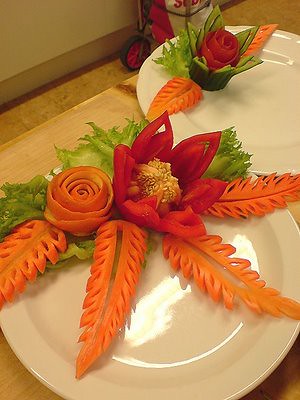The indoor photo captures two meticulously arranged white glass plates on a wooden table, surrounded by a faint suggestion of a gold tablecloth. Each plate features an artistic display of edible flowers created from various fruits and vegetables. On the right plate, a delicate orange rose made from a spiraled apple peel is adorned with two carrot slices sculpted to resemble leaves, accompanied by garnishes of green lettuce. The left plate mirrors this setup but prominently showcases a red rose also crafted from apple peel, alongside a larger, vibrant red flower constructed from bell pepper petals. This plate is further decorated with four long carrot slices fashioned into leaves and small sprigs of lettuce. In the background, a wheeled bag resembling office mail delivery equipment is faintly visible, adding a subtle touch of context to the setting.